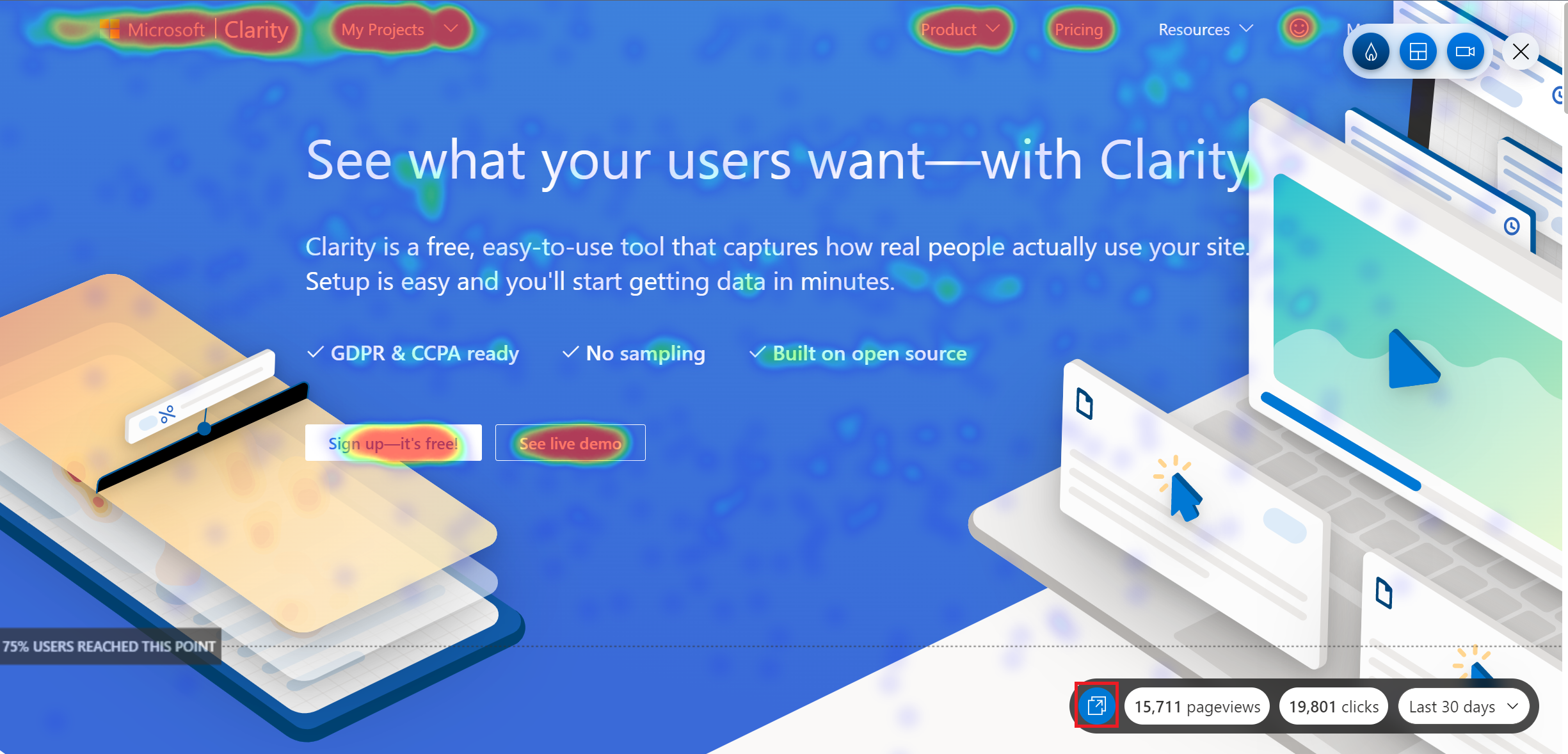The front page of the Microsoft Clarity website presents a distinctive and visually intriguing design, reminiscent of a heat vision effect. This effect centralizes warmer colors like bright orange and transitions to cooler hues such as green and blue towards the periphery.

In the upper left-hand corner, the bold title "Microsoft Clarity" is prominently displayed. Adjacent to this, on the right, is the "My Projects" section, accompanied by a dropdown arrow for additional options. This heat vision styling extends over the "Product" and "Pricing" options next to it, but conspicuously omits the "Resources" option, which instead features a smiley face also adorned with the heat vision effect. Further to the right, there is a submenu offering three distinct icons: a blue circle with a white house silhouette, a blue circle containing a framed silhouette of three squares, and another blue circle depicting an unclear device, followed by an "X" for closing the submenu.

At the heart of the page, a prominent headline reads, "See what your users want with Clarity." It introduces Clarity as a complimentary, user-friendly tool that provides insights into actual site usage, promising a straightforward setup with data collection commencing within minutes. Below this, three check-marked assurances are proudly displayed: "GDPR and CCPA ready," "No sampling," and "Built on open source."

To the right, a dynamic array of images portrays computer screens, user interactions like mouse clicks, and video plays. On the left side, there is a perplexing image resembling a stack of files or documents, paired with an icon that contains a percent symbol. Near the bottom, two buttons are highlighted with the heat vision effect: "Sign up, it’s free" and "See live demo."

At the bottom right corner, a black cylinder-shaped element houses a blue circle enclosed by a red square. Inside this black cylinder are three white circles featuring black text. The first white circle reports, "15,711 page views" and "19,801 clicks in the last 30 days", adding a statistical context to the visual narrative.

Overall, the design not only captivates with its unique visual effects but also effectively communicates the capabilities and benefits of using Microsoft Clarity.